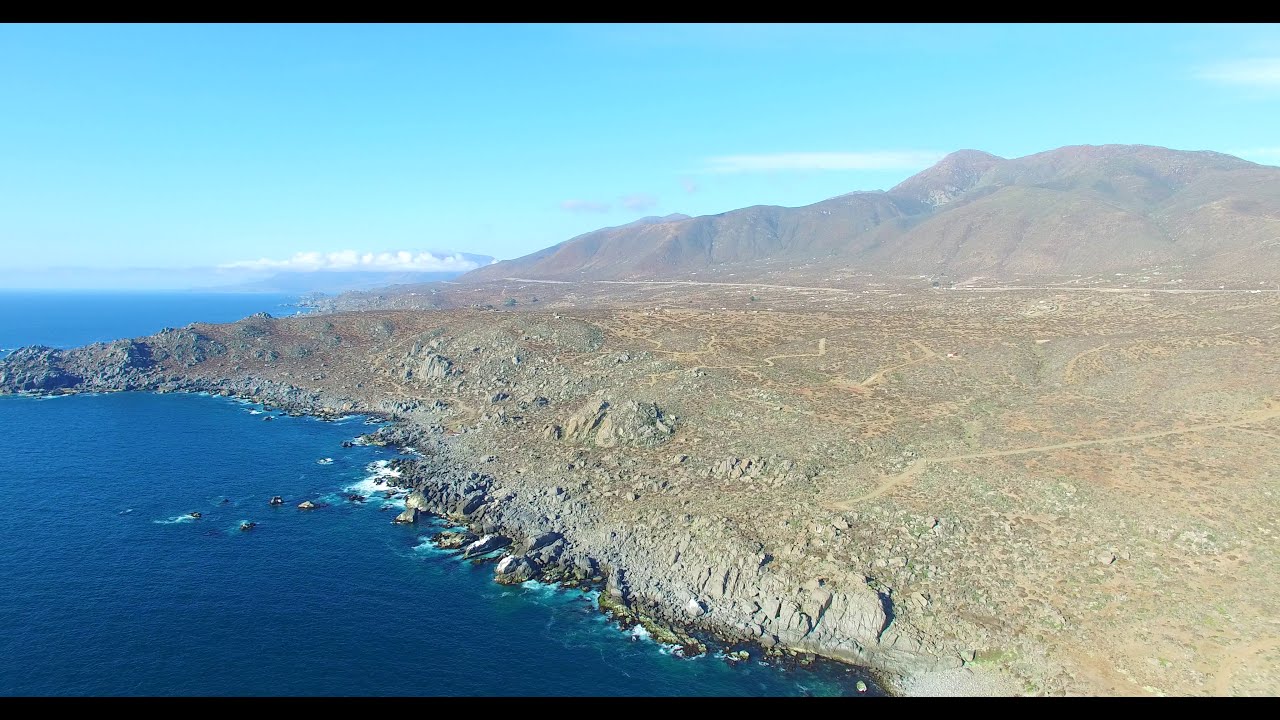This detailed aerial photograph captures a breathtaking coastal landscape from above, showcasing a vivid interplay between land and sea. The serene blue ocean occupies the lower right corner of the image, meeting a rugged, rocky shoreline characterized by steep cliffs and dotted with some random rocks along the curved shoreline, where white foam is visible at the water's edge. This coastal scene gives way to an expansive, monotone gray rocky area that transitions into a majestic mountainous range, rising prominently on the upper right. The landmass extends from right to left, narrowing to a point and featuring a mix of browns, greens from sparse grass, and vast stretches of dirt and rocks. The sky above is a clear, beautiful blue with a few scattered white clouds, enhancing the natural splendor of the landscape. Additionally, a few boats can be seen navigating the clear blue waters, adding a touch of activity to this otherwise serene and untouched panorama. The photograph, likely taken by a drone, offers a high-definition, expansive view of nature in all its glorious detail.